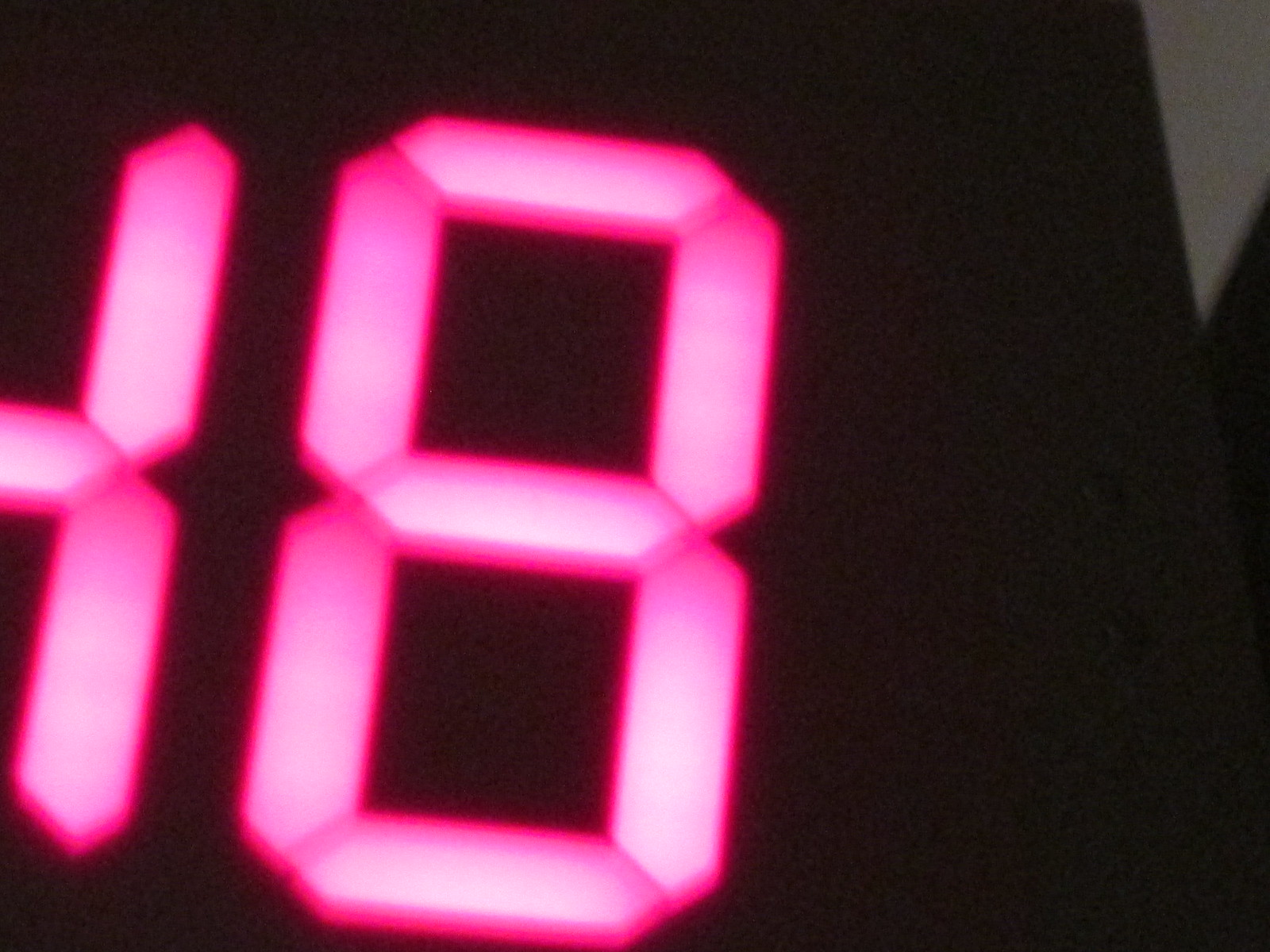This is a close-up photograph that seems to capture the display of a digital clock or timer. The background of the image is predominantly black, with a small patch of dark gray in the top-right corner, which tapers to a point like an upside-down triangle. Central to the image are illuminated numbers: a partially visible number 4 on the left, and a fully visible number 8 to the right. The numbers are composed of segmented parts that are reddish-pink in color, with a gradient that transitions from darker edges to a lighter, almost white center. The 8 is distinctly made up of seven segmented pieces, enhancing its broad and illuminated appearance. The overall effect is a striking contrast of dark and light, with the pink and white neon hues of the numbers standing out against the black background.